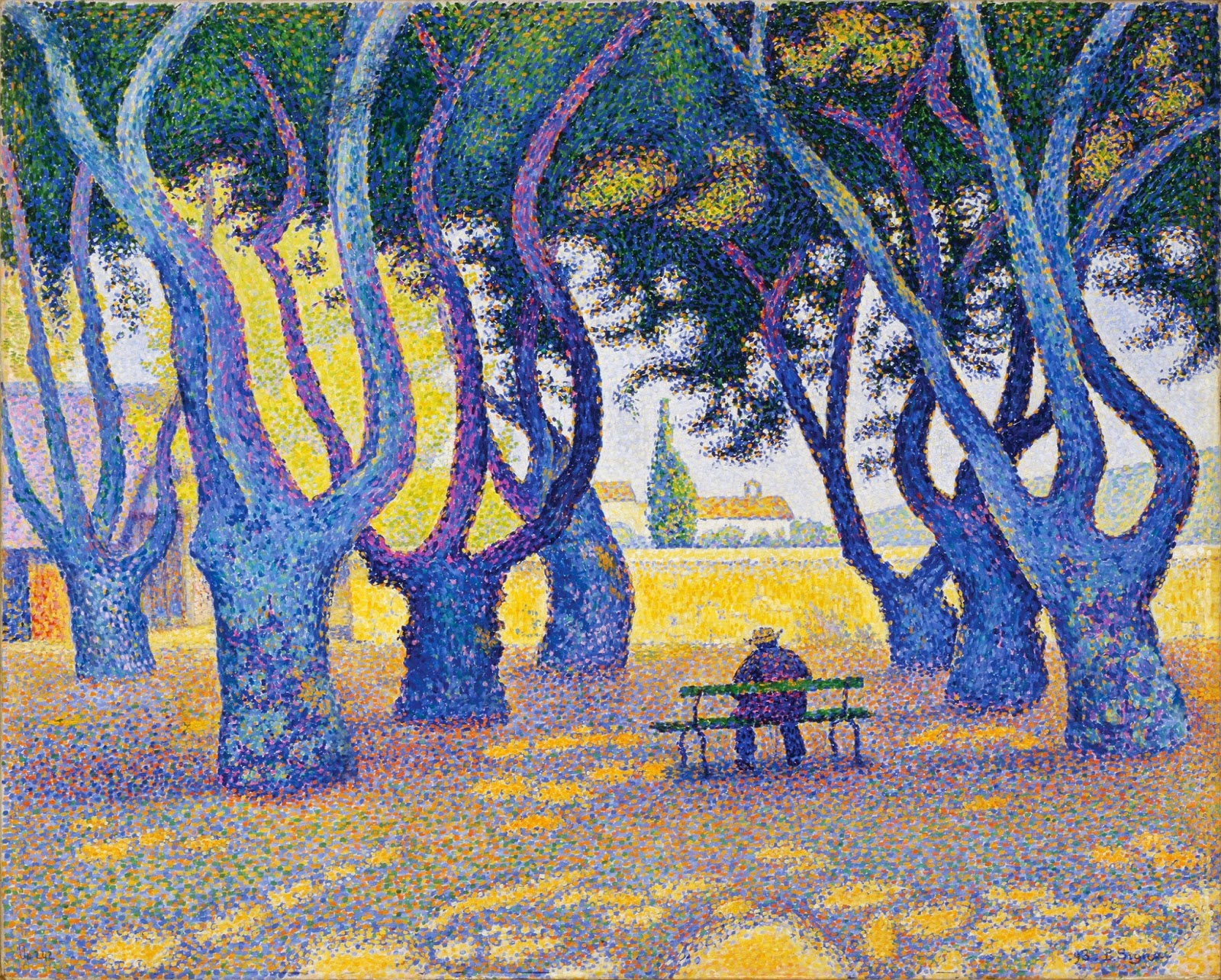This vibrant Neo-Impressionism painting, reminiscent of Van Gogh's style, employs pointillism to create a dynamic, almost psychedelic scene. At the heart of the image, a person donning a beige-yellow hat sits on a green bench. The bench is situated in a field dotted with yellow, purple, and blue spots, adding to the whimsical atmosphere. Surrounding the person are seven massive trees with blue trunks and limbs, some shaded with purplish-pink hues. These trees have tentacle-like branches reaching for the sky, while the canopy above blends greens, yellows, and blues. In the background, a large green bushy tree anchors the scene, with a house featuring an orange roof and chimney positioned to its right. To the left, another structure, perhaps a shack, stands out with its purple roof and orange door. The skyline transitions from white to yellow, completing this richly detailed countryside landscape.